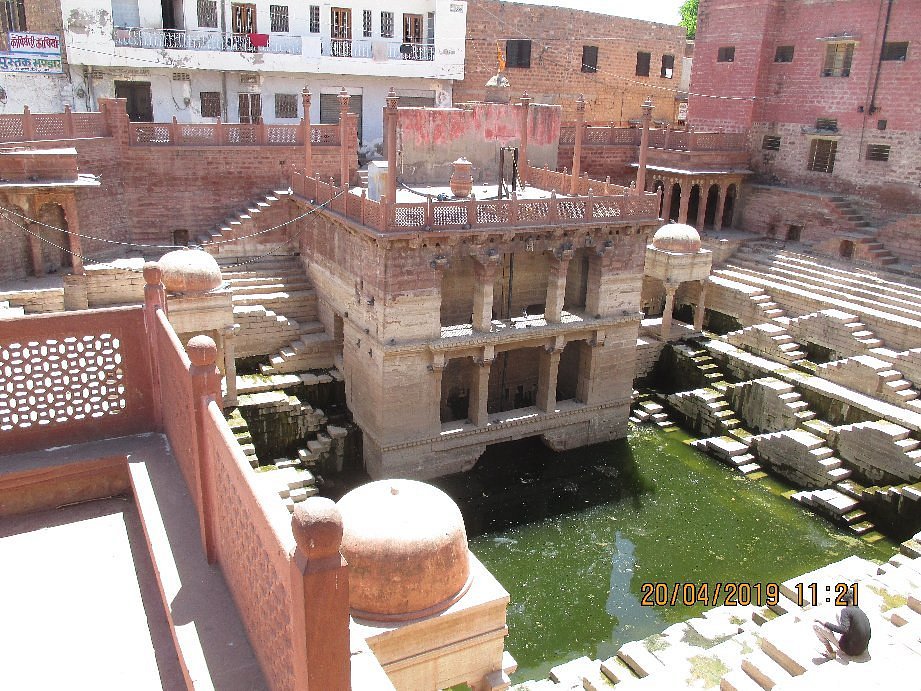This detailed photograph, taken on April 20, 2019, at 11:21 AM, showcases an old, possibly Indian, architectural structure prominently centered over a murky, green body of water. The image, captured in daylight, reveals a series of staircases on either side that descend intricately down to the water level. In the pool's center, there's a distinctive structure featuring windows and a light red railing on top where individuals could stand. On the bottom right, a person is seen seated on the steps, gazing towards the water, with his hand resting on his knee. Surrounding this focal point, the background is filled with a multitude of brick and stone residential buildings in colors of off-white, pink, gray, and black, evoking the atmosphere of a historic, possibly ancient city. The photograph, taken from a higher vantage point, offers a glimpse of the surrounding architectural details, adding depth and a sense of place to the scene.